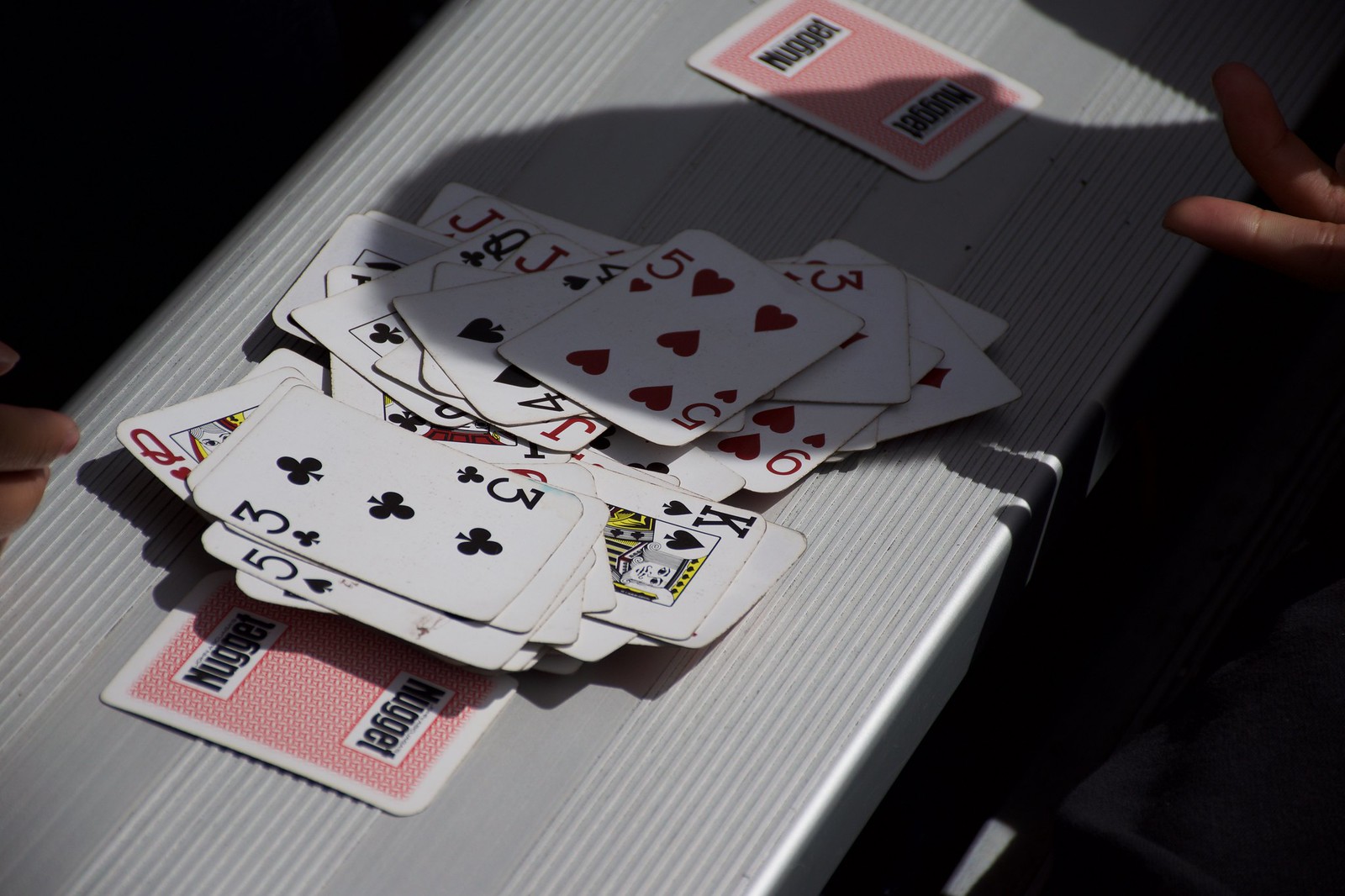This image features a stack of playing cards scattered across a sleek, silver metallic table. Two fingers are visible on the right side, while two additional fingers appear on the left, partially framing the scene. On the right, a flipped card displays the word "Nugget" in black letters within a white box; this card has a red backing with a white frame. Towards the left, closer to the central pile, another card also bearing the word "Nugget" lies visibly. 

At the heart of the image, a disorganized pile of playing cards is strewn across the table. The cards are laid out haphazardly, revealing their faces to the viewer. Among them, distinct cards can be identified: the five of hearts, the three of clubs, the king of spades, the nine of hearts, the jack of an unspecified red suit, the queen of hearts, and the five of spades. The entire arrangement of cards is reminiscent of leaves being gathered together in the fall, creating a sense of casual disarray. Additionally, two cards are face down, their identities hidden from view.